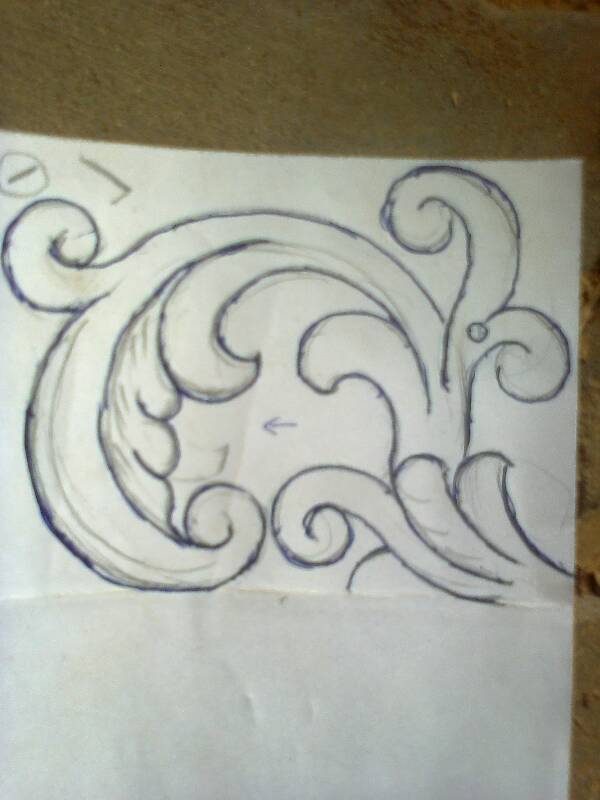A meticulous pen drawing on plain paper depicts an intricate wave, though it also carries a resemblance to a stylized emblem or a fleur-de-lis. Instead of presenting as a uniform mass, the wave is composed of elaborate, appendage-like extensions that curl and twist upon themselves. These delicate tendrils seem to capture the dynamic movement of water moments before they cascade downward, creating a sense of imminent fluid motion.